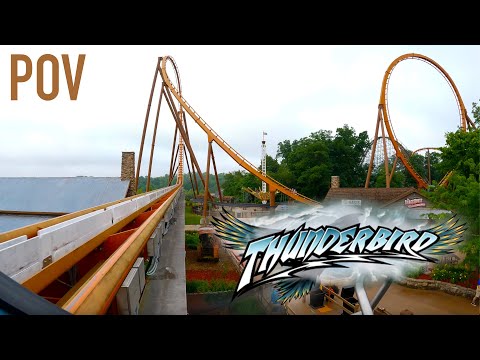The image captures an outdoor scene at a theme park, framed with black bars at the top and bottom, possibly indicating a video thumbnail. Dominating the foreground, an orange roller coaster track of the Thunderbird ride loops dramatically amidst a backdrop lush with green shrubs and towering trees. On the left side of the image, a partial view of a house rooftop peeks through the greenery. In the top left corner, bold orange letters spell out "P.O.V.", while the bottom right corner features the word "Thunderbird" in large block letters that transition from teal to white, complemented by teal wings with yellow tips extending from either side. Additionally, behind the text, there's a cloudy mist and a jagged lightning bolt extending from the final "R" in "Thunderbird". From this vantage point, it is clear that the perspective is from the front row of the roller coaster, capturing part of the vehicle and the dynamic loops of the track, with hints of other theme park attractions and walkways visible in the background under a grey, cloudy sky.